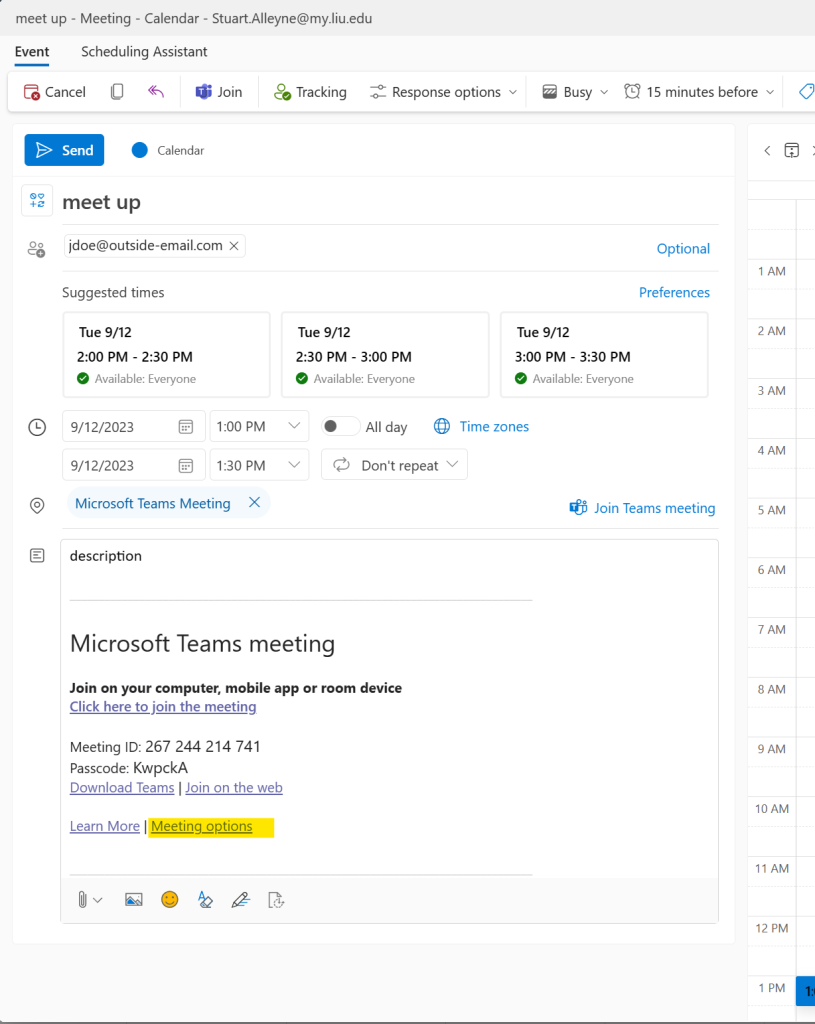This image, sourced from a website, showcases a streamlined online meeting interface. At the top, a light gray background hosts the black text "Meetup Meeting Calendar" accompanied by an email address. Below, the background transitions to white, featuring the word "Event" in black with a blue underline. Adjacent to "Event," the label "Scheduling Assistant" appears.

Following this, there is a horizontal row of options: "Cancel," "Tracking," "Response options," and "Busy 15 minutes before," culminating in a blue box labeled "Send." Beside the "Send" button, a blue circle with the word "Calendar" is present.

Highlighted below these controls are suggested meeting times, all labeled "Tuesday 9-12," with specific slots: 2:00 PM to 2:30 PM, 2:30 PM to 3:00 PM, and 3:00 PM to 3:30 PM. Below the suggested times, there is a text box available for input. The page concludes with a horizontal black line running across the bottom, marking the end of the interface.